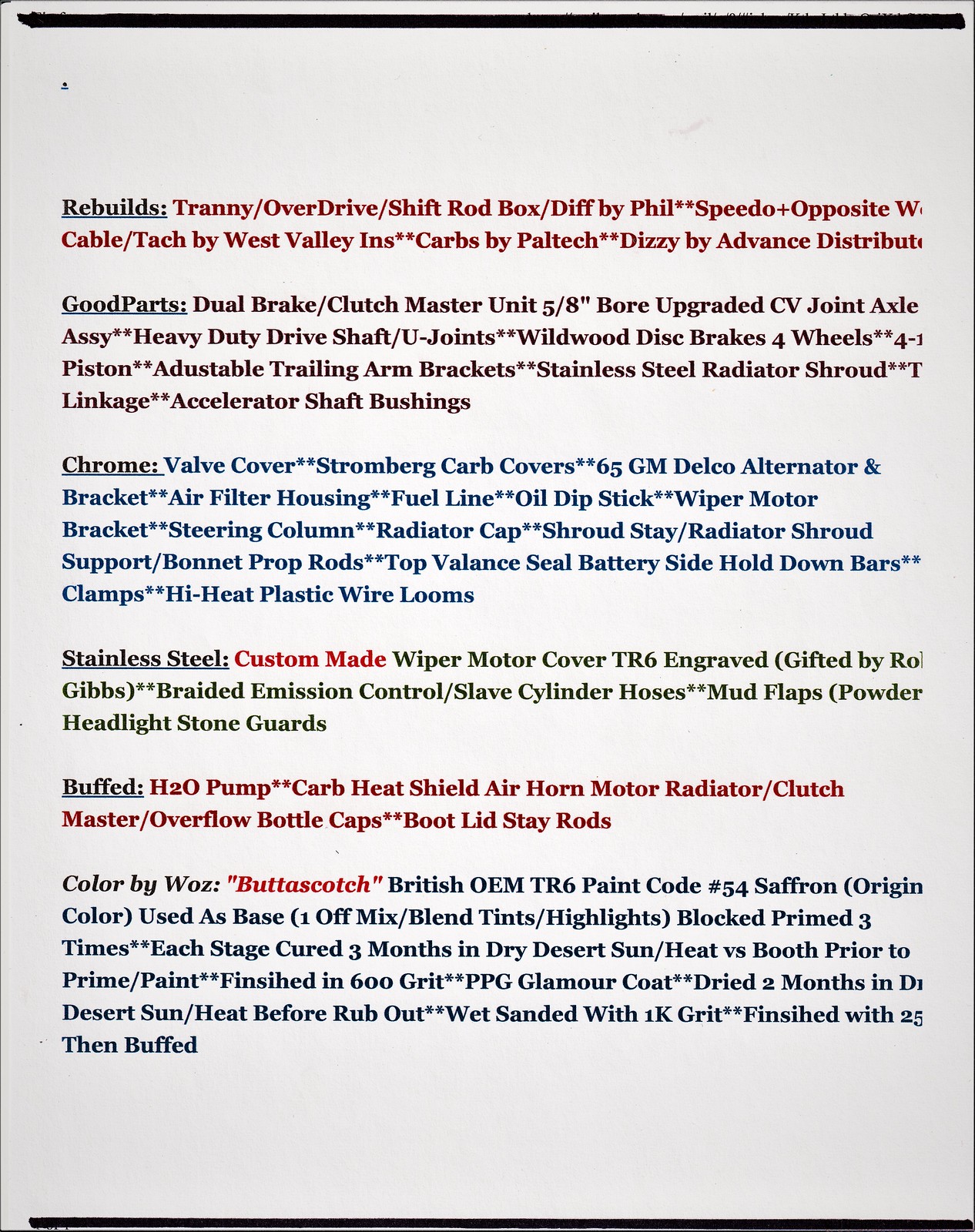This detailed image depicts a meticulously organized reference sheet on a white background, bordered by a black line at both the top and bottom. The sheet contains a comprehensive list of terms divided into six categories: Rebuilds, Good Parts, Chrome, Stainless Steel, Buffed, and Colored by Woz. Each category, highlighted in distinct colors, lists various components and their specific details. 

Under **Rebuilds**, notable items include "Tranny/Overdrive/Shift Rodbox" in red, "Diff by Phil," "Speedo + Opposite W. Cable/Tech by West Valley Inns," and "Carbs by Pal Tech." There's an emphasis on red-lettered specifics such as "Dizzy by Advance Distributed."

In the **Good Parts** section, you find "Dual Brake," "Clust Master Unit 5/8," "CB Joints," "Axle Assembly," "Heavy Duty Drive Shaft/U Joints," and "Wilwood Disc Brakes - 4 wheels, 4, 1 piston." This segment continues with "Adjustable Trailer Arm Brackets," "Stainless Steel Radiator," and "Accelerator Shaft Bushings."

For **Chrome** items, the image lists "Valve Cover," "Stromberg Carb Cover," "65 GM Delco Alternator and Bracket," "Air Filter Housing," "Fuel Line," "Oil Dipstick," "Wiper Motor Bracket," "Radiator Cap Shroud," "Bonnet Props," and "High Heat Plastic Wire Looms."

In the **Stainless Steel** section, the emphasis is on custom-made items such as "Wiper Motor Covers TR6 (Engraved by Roe Gibbs)," "Braided Emission Control/Slave Cylinder Hoses," "Mud Flaps," and "Headlight Stone Guard."

The **Buffed** category includes "H2O Pump," "Carb Heat Shield," "Air Horn Motor," "Radiator/Clutch Master," "Overflow Bottle Caps," and "Boot Lid Stay Rods."

Lastly, for the **Colored by Woz** category, identifiable items include "Butterscotch" and "British OEM TR6 Paint Code #54 Saffron," used as a base mix for blending. It describes a meticulous finishing process involving "Block Prime three times," with each stage cured for three months in dry desert sun, followed by heat reverse boost prior to final prime/paint with a "600 grit PPG Glamour Coat," dried for two months before being "wet sanded with 1K grit, and finished with 25, then buffed."

This sheet serves as a comprehensive guide where one can select and customize parts based on exact specifications and preferences.